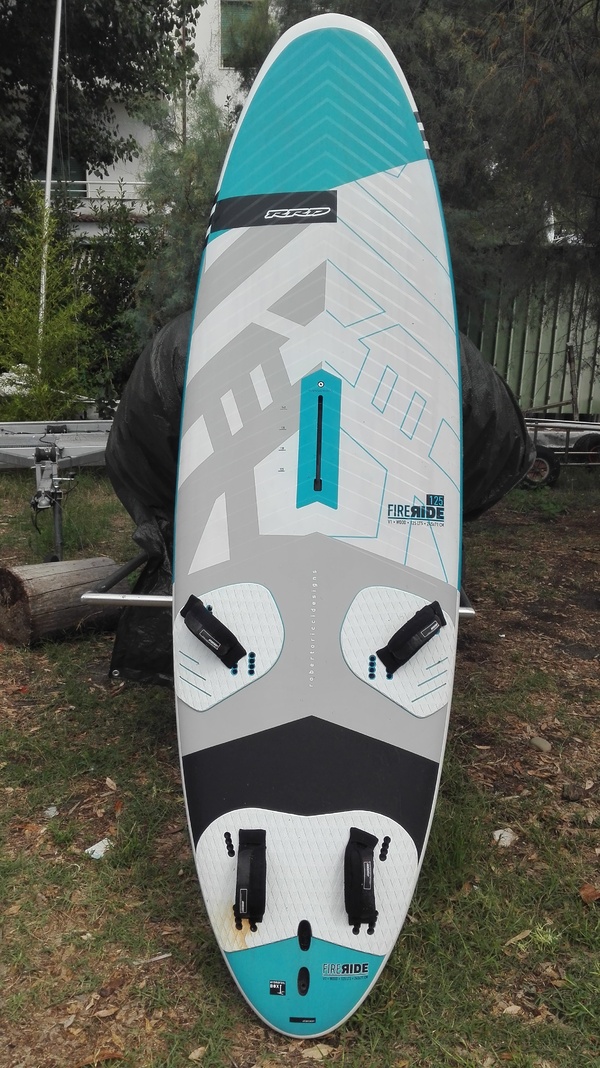The image depicts a light blue surfboard or paddleboard leaning upright against the tire of a boat trailer in a grassy backyard. The board features a predominantly pale silver-gray background with blue highlights at the top and bottom, as well as black and gray patterns. Four black straps for securing feet are visible, and a hole in the center is designed for attaching a keel. The brand name "Fire Aid" is written just below the center on the right-hand side. Surrounding the board, there is yard debris including a wooden log, a green metal storage shed on the right, and potential trailers on both sides. A vine-covered chain link fence and trees are also seen in the background, suggesting a residential area with possibly an apartment building or house in the distance.